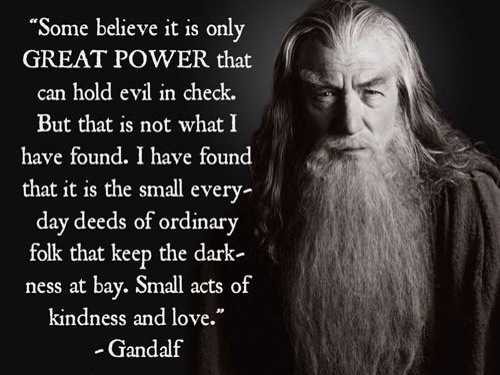The image features a black-and-white still of Sir Ian McKellen portraying Gandalf from The Lord of the Rings. Positioned on the right side, Gandalf is seen wearing a plain black robe, with his long white beard and hair framing his face. He gazes directly at the camera with a serious expression against a plain black background. On the left side of the image, in a white Times New Roman font, is a motivational quote: "Some believe it is only great power that can hold evil in check, but that is not what I have found. I have found that it is the small everyday deeds of ordinary folk that keep the darkness at bay, small acts of kindness and love." This layout suggests the image is either a screenshot or a meme, intended for inspirational sharing on social media.